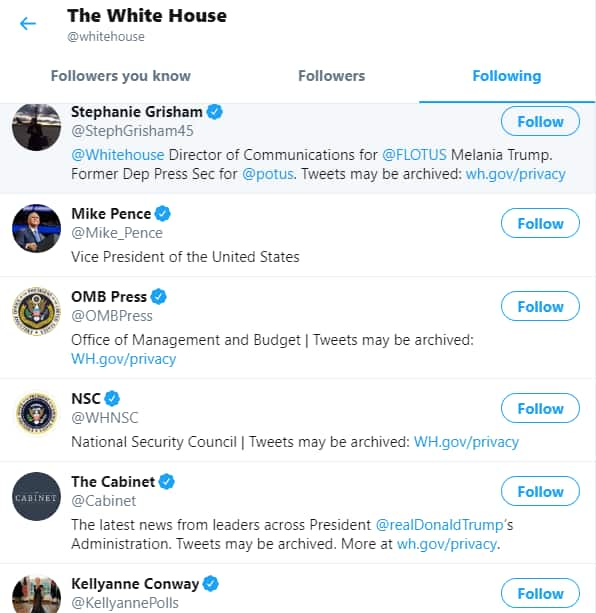This is a detailed screenshot of a Twitter page showcasing the "Following" list of the official White House account, highlighted in blue. The screenshot is taken during Donald Trump's presidency. The first profile on the list is Stephanie Grisham, distinguished by a verified blue tick. Following her is the account of Mike Pence, noted as the Vice President of the United States at the time. Next on the list is OMB Press, the official Twitter handle for the Office of Management and Budget. This is followed by the NSC, the handle for the National Security Council. Further down, the account for the Cabinet is displayed, providing news updates from various leaders within the President's administration. Lastly, the screenshot shows that the White House account is following Kellyanne Conway's profile.